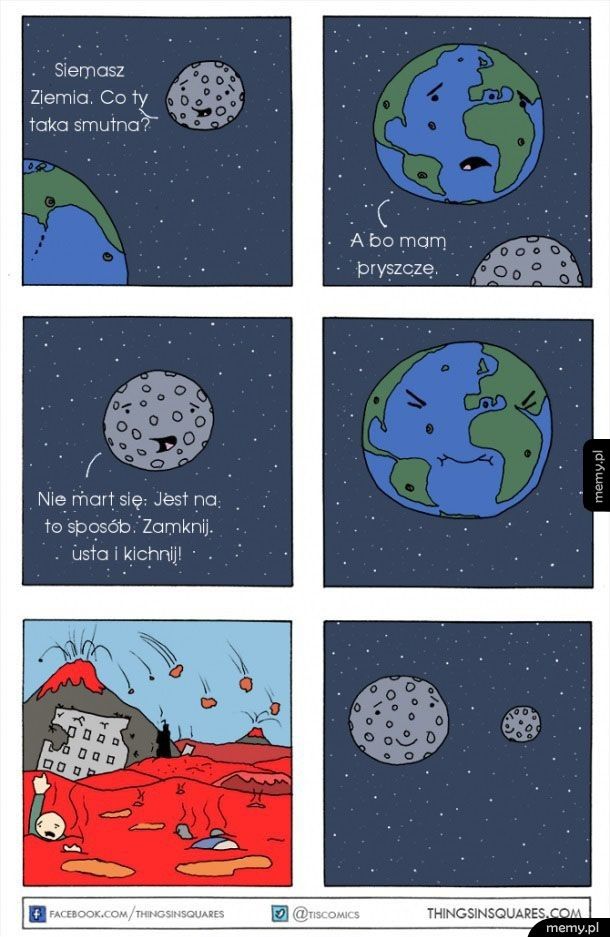In this composite image of six digitally created illustrations, arranged in three rows with two images per row, we are presented with a series of scenes that have a comic-style aesthetic, likely intended for social media sharing. 

The first four images depict a whimsical, interplanetary dialogue between the Earth and the Moon. In the first image, positioned in the bottom left corner, we see the Earth conversing with the Moon, which has a small mouth facing the Earth. The Moon appears to be speaking in a language that is not immediately recognizable. In the second image, Earth is centered with expressive eyes and a speaking mouth, while the Moon is in the lower right. The third slide focuses solely on the Moon, which seems to be engaged in a monologue, presumably directed at Earth. The fourth image captures Earth alone, making a scrunched face that suggests it is either reacting to something unpleasant or experiencing discomfort, as if it had been kicked or tasted something sour.

The fifth image takes a dark turn, depicting a chaotic apocalyptic scene with a volcano erupting violently. Amidst the fiery landscape, people are seen swimming and sinking into streams of molten lava, amplifying the sense of turmoil and destruction. 

The final image returns to a cosmic theme, showing two moons floating in the vastness of space. The color palette throughout the series features dark blue, gray, green, light blue, red, orange, and different shades of green, contributing to the vibrant yet contrasting atmospheres depicted in each frame.